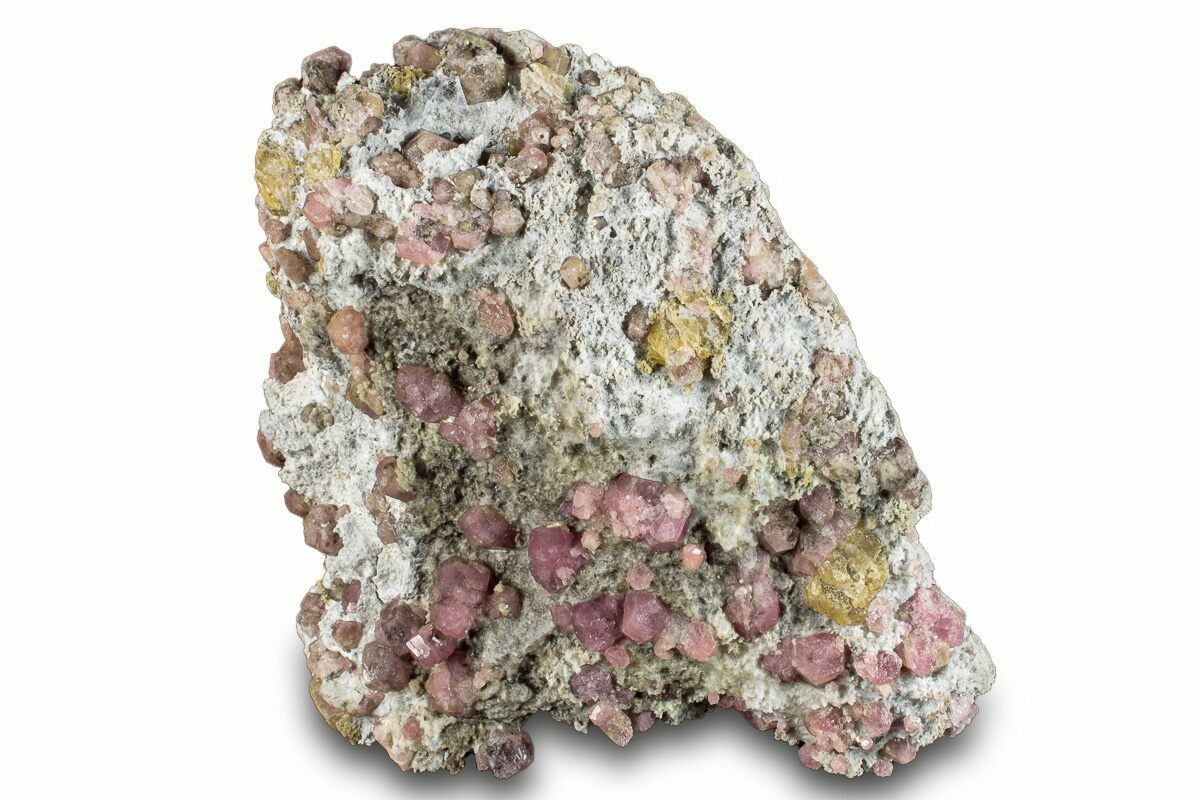This is a detailed, full-color photograph of a rough, unpolished rock, prominently featuring a variety of minerals and crystals. The image is staged against a plain, white background with some shadowing at the bottom, and shows a jagged, uneven, and roughly textured rock. The rock stands about 8 to 10 inches tall and has an irregular shape, somewhat resembling an oval or circle but with bumpy and lumpy dimensions. The base color of the rock is a light gray, and its surface is studded with an array of colorful, embedded minerals.

Scattered across the rock are numerous light pink or mauve crystals, as well as patches of medium yellow and shades of gray or light brown. The colors vary from pale grays and purples to yellowish-greens, giving the rock a strikingly diverse appearance. The pink crystals appear to be particularly fragile, almost as if they could be picked off with a needle or small tool. Despite the rock's overall gray base, most of its surface is covered with these colorful mineral inclusions, providing a vivid contrast against the coarse, porous texture.